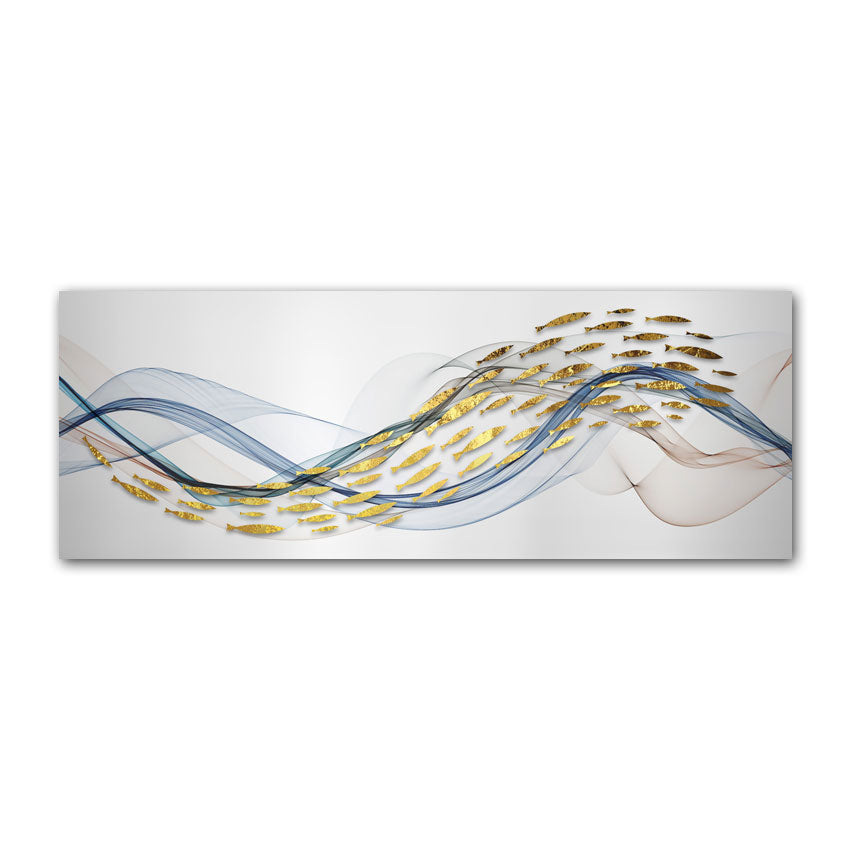The artwork is an intricate, rectangular piece displayed on a white surface. Dominating the soft gray background are airy, sheer swirls reminiscent of tulle fabric, in soft aqua, blue, deeper blues, and bronze hues. These swirls, resembling gauzy ribbons, stretch from left to right, varying in thickness and detail. Overlaying this delicate backdrop is a pattern of small, golden fish, subtly blending into the artwork. The fish appear to follow the undulating bands of color in a wave-like formation, almost reaching the right edge. Although abstract in nature, these elements together give an impression of fish swimming through the rhythmic motion of ocean waves, creating a compelling, visually appealing scene despite the absence of a visible signature.